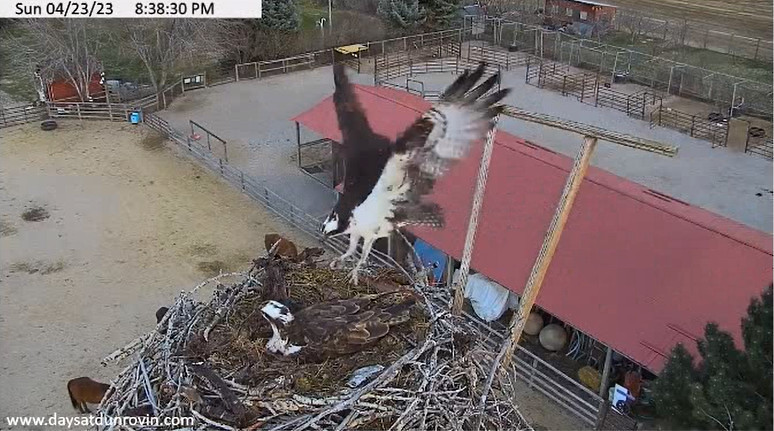The security camera image captures an impressive scene of avian activity at a ranch, identified by the website www.daysatdunroven.com in the bottom left corner. The timestamp on the top left corner reads Sunday, April 23, 2023, 8:38:30 PM. The camera, mounted high up, overlooks an expansive outdoor pen surrounded by fences and various smaller pens with steel cages. Dominating the foreground is a meticulously constructed bird's nest made of twigs, positioned slightly left of center along the bottom of the frame. 

The nest is alive with activity as a majestic bird, resembling an eagle with brown feathers and a white head speckled with brown, is about to land. Its wings are fully outstretched, feet extended, and head angled downwards in a precise landing motion. In the nest, another bird of similar appearance is either nesting some eggs or attending to young ones, suggesting a familial interaction.

The background reveals a broad view of the ranch, including a large brown building, several outdoor stalls, and the distinct red roof of a barn. The dirt-covered ground and the partially visible horse enhance the rural setting's authenticity. Tall trees border the horizon, adding depth to this dynamic and detailed wildlife photograph.